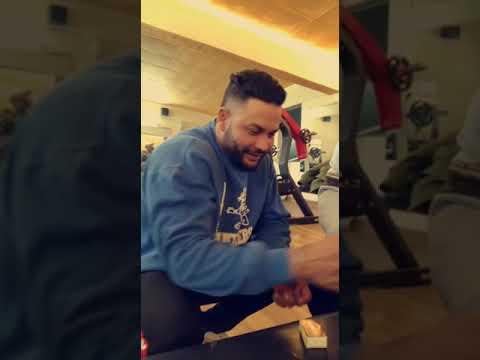In the center of a three-part image, a man is seen kneeling in what appears to be a gym, surrounded by darker, zoomed-in versions of the main picture on either side. He has short, dark brown hair and a small beard with a mustache. The man is wearing a black or possibly blue sweatshirt with white logos and lettering on the front, and black pants. The gym setting features various pieces of workout equipment, including free weights attached to a bar and a bench press or overhead press, colored red, gray, and black. Behind him, the room is filled with gym accessories and machines, and the ceiling has tan beams with a yellowish hue towards the background. He is positioned in front of a dark-colored table on a light brown hardwood floor with visible wood grains.